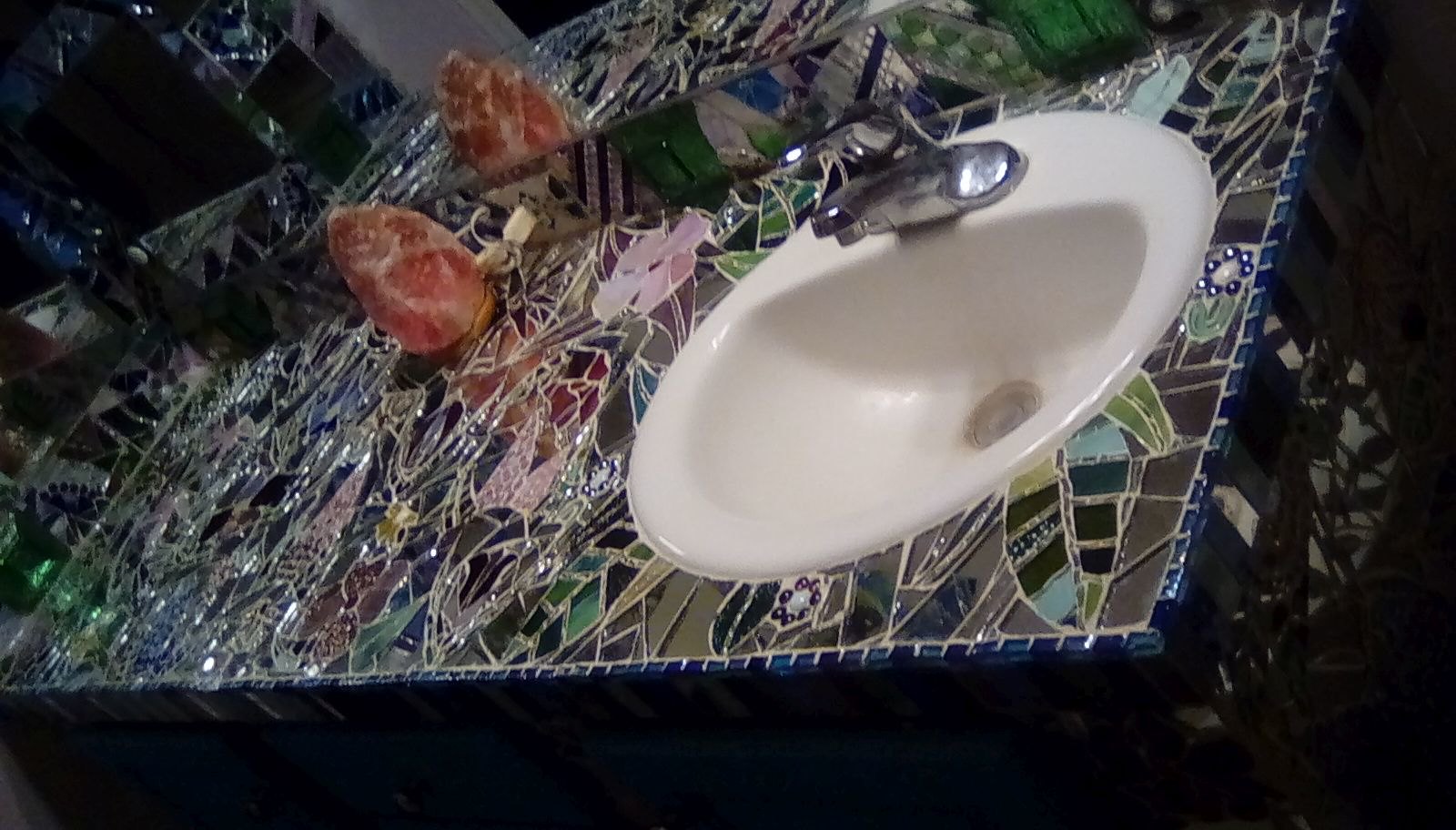This vibrant and captivating bathroom countertop is an extraordinary example of glass mosaic artistry. The lengthy surface is crafted from fragments of colorful glass pieces, intricately arranged to create a stunning, almost stained glass-like appearance, yet it is distinctly mosaic with white grout. Both the left side splash and back splash seamlessly match the countertop, further enhancing its cohesive and artistic appeal.

The mosaic is adorned with floral and leaf designs that sparkle brilliantly due to the reflective nature of the glass. The edge features a mesmerizing array of vertical rectangular glass pieces in varying shades of blue and white, adding a striking border to the intricate mosaic pattern. A pink Himalayan salt lamp is plugged into an outlet set into the back splash, casting a warm glow that complements the countertop’s dazzling colors.

Amidst the vibrant glasswork, a pink flower and a pair of green glass leaf designs add a touch of nature to the artistic tableau. Another larger leaf design incorporates a diverse palette of green, brown, blue, and black glass pieces, showcasing the creator’s skill and creativity. 

Despite the luxurious artistry of the countertop, it features a stark contrast with a basic white sink and an unremarkable single-handle chrome faucet, suggesting that the artisan invested more in creativity than in high-end fixtures. Above the backsplash, a mirror reflects the breathtaking mosaic, doubling the visual splendor of this remarkable work of art. This countertop is truly an exceptional and inspiring focal point in the bathroom.